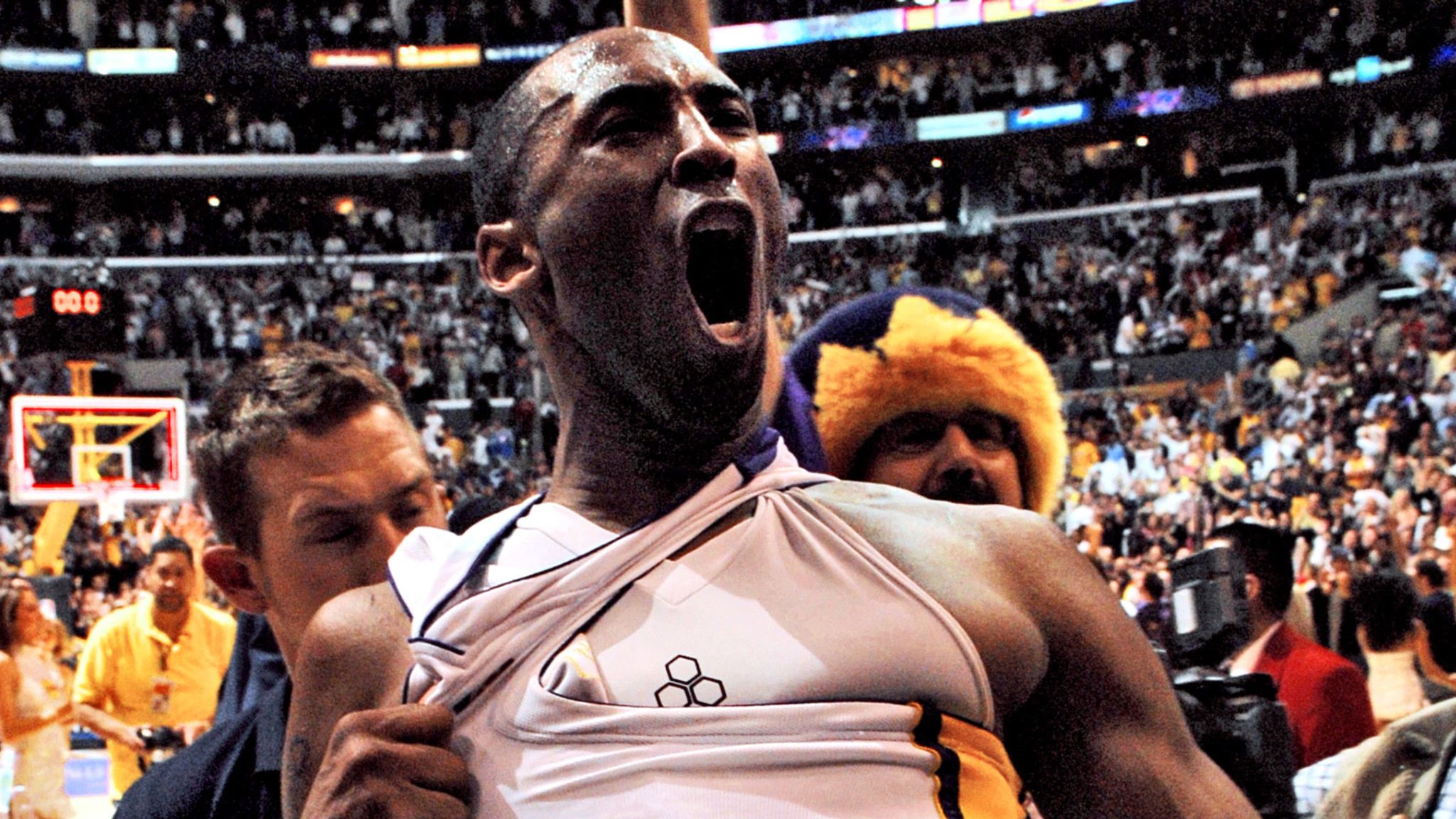In this image, a jubilant Kobe Bryant is captured in the throes of celebration, likely after a significant basketball victory. He is wearing a white Lakers jersey with yellow and black trim, and beneath it, his undershirt is emblazoned with three hexagons arranged in a triangular formation. His expression is one of exuberance, mouth wide open as if yelling or cheering, and his gaze is directed to the right of the viewer. 

Bryant is depicted pulling on his jersey, possibly displaying his undershirt's design in his moment of triumph. Behind him are two individuals—one man with black hair in a black suit and another wearing a distinctive hat resembling a gold-trimmed crown with a black top. Further in the background, you can see the bustling basketball court on the left, complete with a basketball hoop and a shot clock displaying zero seconds. The arena is packed with a multitude of spectators, many adorned in yellow, their energy palpable. Cameras are also visible amidst the crowd, capturing the electrifying atmosphere. Above the audience are rows of advertisements and box seats, encapsulating the high-stakes environment of a pivotal basketball game.